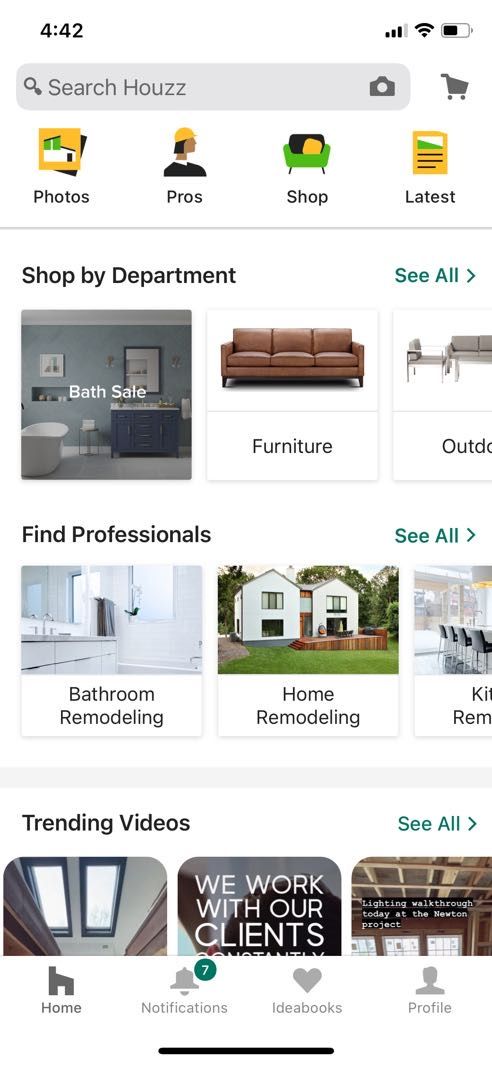This digital screenshot showcases a shopping interface on a home improvement website. On the left side, the 'Shop by Department' section features a prominent banner for a Bath Sale, displaying a large white bathtub, a sizable bathroom mirror, a blue cabinet, a chair, and wall-mounted light fixtures. To the right, under the furniture category, there's an image of a large brown couch with three bottom cushions and three back cushions. The interface includes a 'Home Remodeling' button, accompanied by an image of a well-maintained home with a lush green lawn. Also visible are buttons for 'Photos', 'Pros Shop', and 'Latest', as well as a small shopping basket icon.